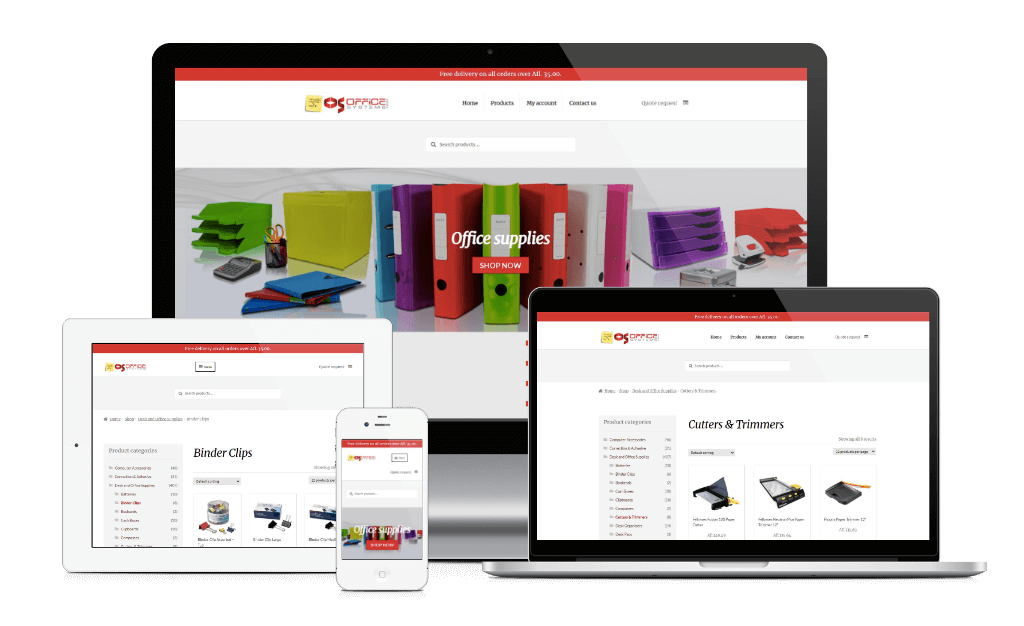This vibrant advertisement features a range of office supplies displayed across various devices, emphasizing a unified shopping experience. In the background, a large monitor prominently showcases a webpage titled "OS Office," with a bold "Shop Now" button in red. The webpage's main banner reads "Office Supplies" and displays images of multicolored folders — in hues of red, purple, blue, green, white, and pink — alongside a diverse arrangement of office essentials such as a calculator, various file holders, and a pen holder containing orange scissors.

To the left, a tablet exhibits a slightly blurred section but clearly mentions "Binder Clips." Below this, the tablet screen mirrors the monitor’s main page. Positioned centrally, a smartphone screen replicates the office supply banner seen on the monitor, ensuring continuity across devices.

On the right, a smaller laptop screen highlights a different webpage section focusing on "Cutters and Trimmers," featuring images of three black paper cutters with distinctive yellow trims. This carefully arranged visual advertisement underscores the variety and accessibility of office supplies available for purchase across multiple devices, enhancing user convenience and engagement.